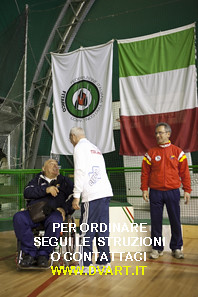This vertically aligned rectangular photograph appears to be taken inside a gymnasium. In the background, two flags are prominently hung. The flag on the right features horizontal stripes of green, white, and red from top to bottom. To its left hangs a white flag with a green circular emblem that encompasses a white center and a red icon in the middle, although the specifics and surrounding text are indistinguishable due to distance. The gymnasium's roof is constructed of a green vinyl tarp-like material supported by an ascending metal arch in the upper left corner.

In the foreground, three men are positioned centrally. On the right stands a man in his 50s with short gray hair and glasses, dressed in a red jacket with yellow and white stripes on the sleeves, blue jeans, and tennis shoes. In the middle, an elderly man in a white jacket and blue track pants leans down to shake hands with another elderly man in a wheelchair on the left. The man in the wheelchair is clad in a blue leisure suit, consisting of a casual exercise jacket and pants. A green metal fence is visible behind them. At the bottom of the image, yellow text reads "Perord, Nair, Seguil, Struzion, O. Contatosi" along with the website "www.dvar.it," indicating likely foreign language content.